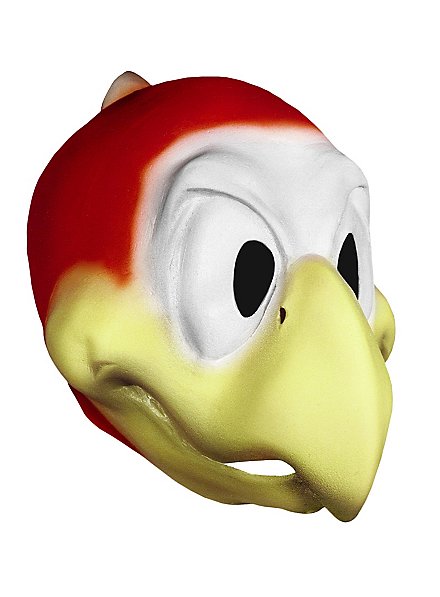This photograph showcases a vividly colorful, cartoonish Halloween mask resembling a duck's head. The mask is three-dimensional, potentially made from ceramic or created through a computer design. The head is predominantly red on the top and back, with a small stump-like protrusion at the rear, possibly representing a feather. The area around the eyes and forehead is white, punctuated by black pupils centered within the eyes. The beak and mouth, extending to the cheeks, are painted a vibrant yellow. There is a visible nose hole on the beak's left side. The photograph is square, approximately four inches by four inches, set against a plain white background, with no additional identifying details regarding the time, location, photographer, or mask creator.